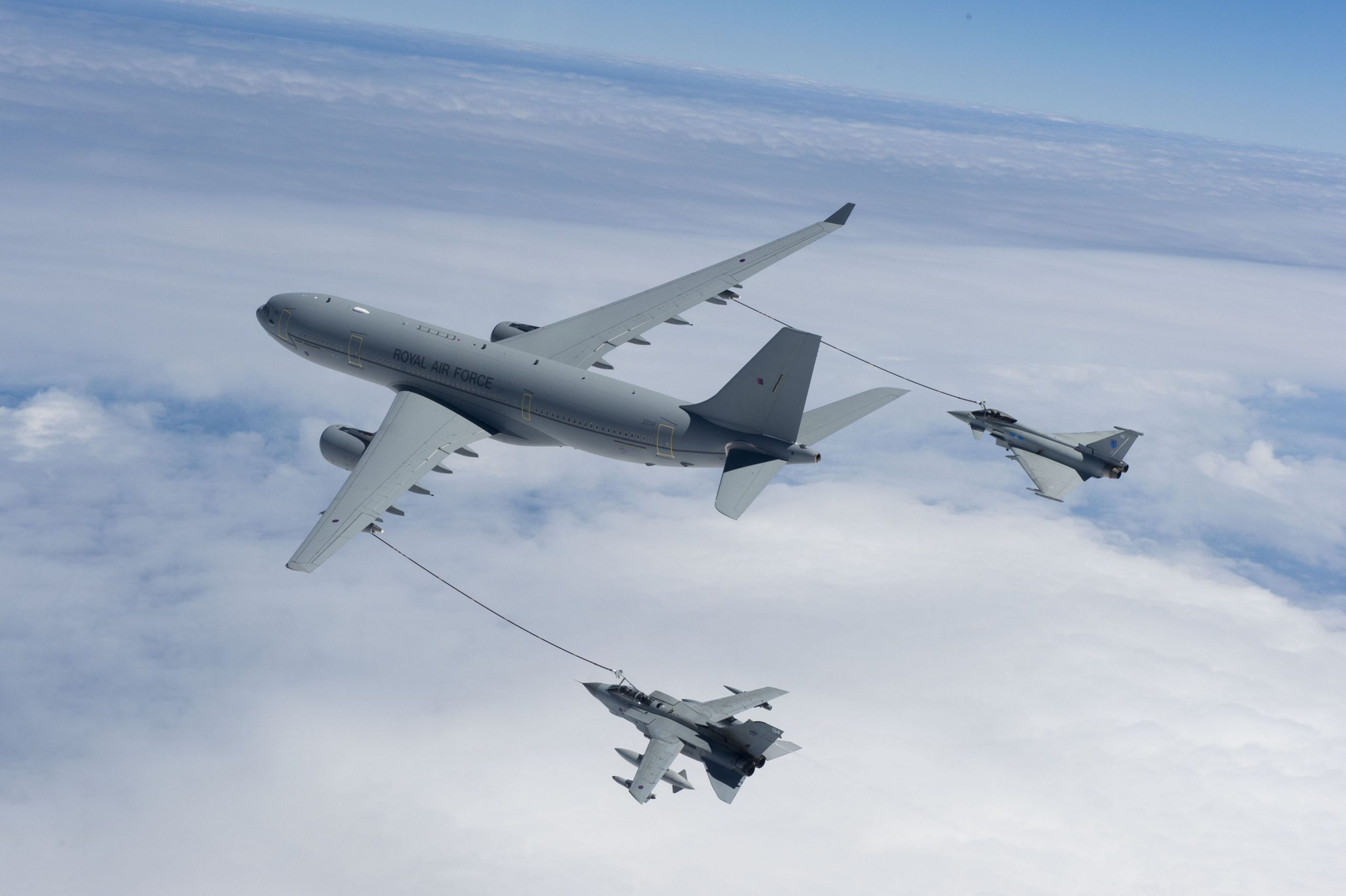This image, taken high up in the sky, features three grey aircraft above a blanket of white clouds with a patch of blue sky visible in the upper right corner. The central and largest plane, identified by its black lettering as part of the Royal Air Force, is a refueling aircraft. It extends fuel lines from both wings to two smaller fighter jets positioned on either side. The jets are also grey and are equipped with bombs. The refueling plane is silver or grey and the scene vividly showcases the intricate mid-air refueling operation against a backdrop of beautiful blue and white hues.